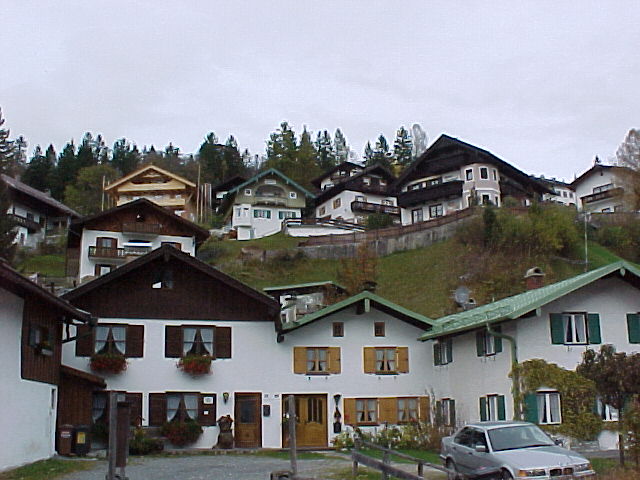This image captures a scenic hillside dotted with houses and cottages, primarily resembling resorts or hotels, but potentially serving as residential buildings. The structures are arranged in three distinct rows ascending the slope, resembling Hollywood’s hillside homes, or European chalets. At the forefront, a large white multi-family residence or inn dominates, featuring several gables and contiguously connected sections. The building showcases a mix of green, black, and yellow sloped rooftops, brown shutters, and open windows adorned with white curtains. A grey car, identified as a BMW, is seen emerging from the middle portion, heading towards the right. Further up the hill, standalone two-story houses of similar architectural style, but varying in roof color, are interspersed among the verdant green grass and characteristic coniferous trees. The background features a row of pointy, conically shaped evergreen trees under an overcast sky, hinting at possible rainfall, yet the daylight suggests a serene, picturesque setting.